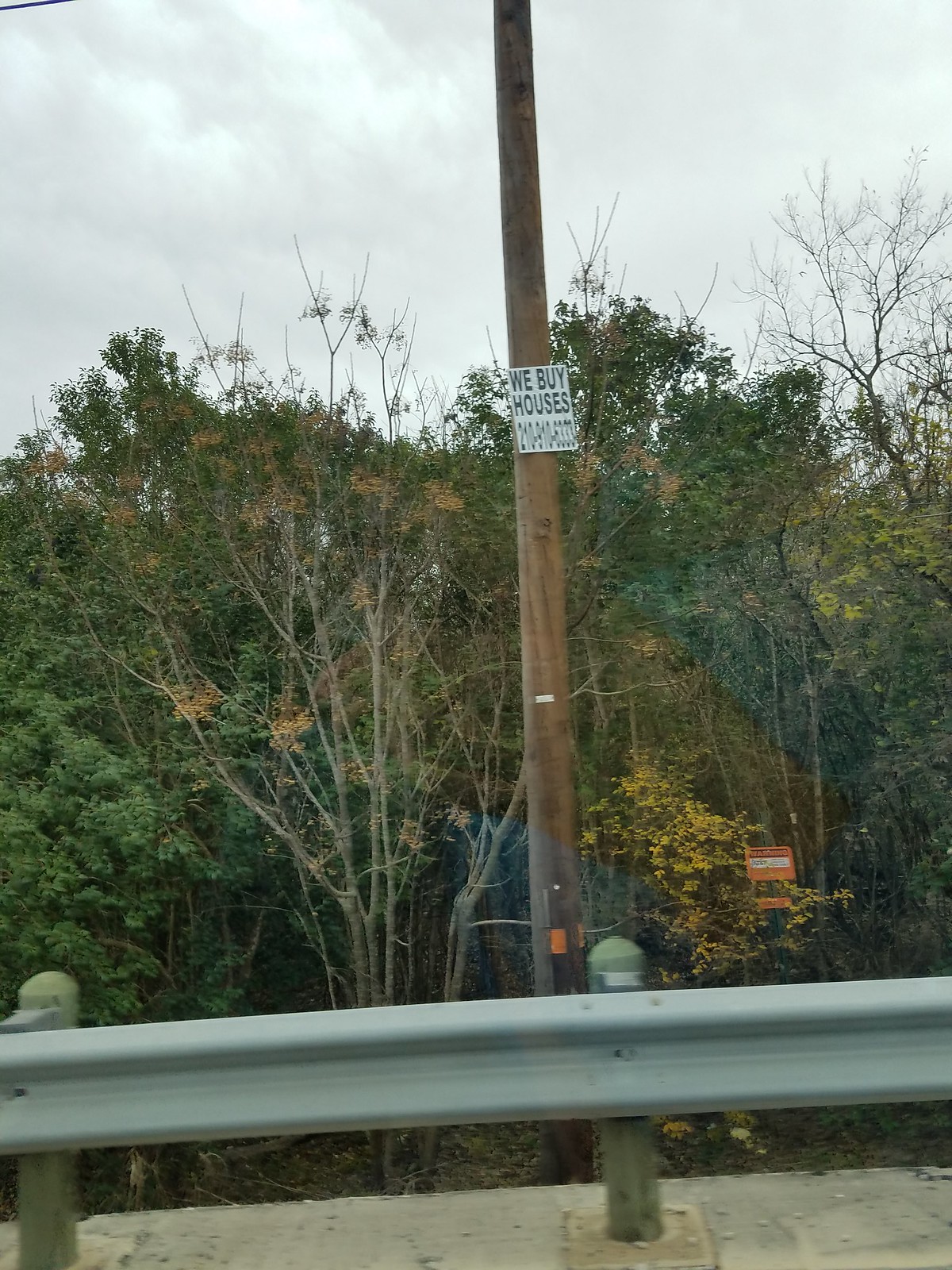The photograph captures the edge of a roadway, prominently featuring a gunmetal-colored steel guardrail riveted to pegs emerging from a concrete pathway. Just beyond the guardrail, a tall brown wooden pole stands with a white sign midway up that reads "We Buy Houses" in black text, accompanied by a phone number at the bottom. The pole is set against a backdrop of a wooded area; the trees in the foreground are bare, while those in the background are densely leaved, suggesting a seasonal transition. The sky above is overcast and gray, with a hint of sunlight peeking through the upper left corner, further insinuating an autumn setting. The photograph appears to have been taken from inside a vehicle, as evidenced by a subtle reflection on the glass window. The ground below the roadway drops down to a lower level, creating a slight elevation difference between the road and the forested area.